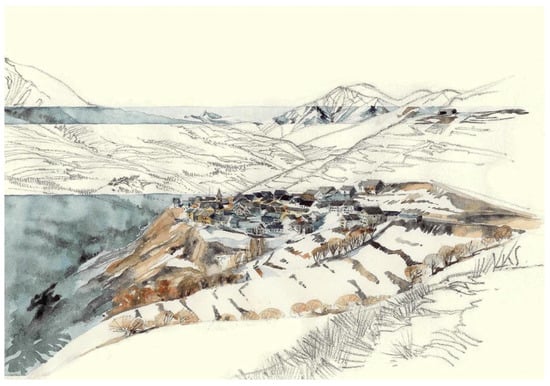This watercolor image depicts an alpine village nestled amidst snow-covered mountains. At the base of the artwork, there is a section with basic line work representing grass, creating a simple foreground. Slightly above this, the mountainous region is more detailed and colored, featuring snow-capped peaks and rugged paths. In the middle of the image, a cluster of small buildings, possibly traditional village houses, sits on a plateau, surrounded by snow and dotted with trees. A cliff drops into an abyss beside the village, accentuating the dramatic landscape. The background consists of more intricate line work of mountains, with patches of visible grass and brown rock breaking through the snow. The sky seamlessly blends into the snowy peaks, making it challenging to distinguish where the snow ends and the sky begins, as both are rendered in a uniform white texture. This image evokes a sense of nostalgia, reminiscent of illustrations from a childhood textbook.